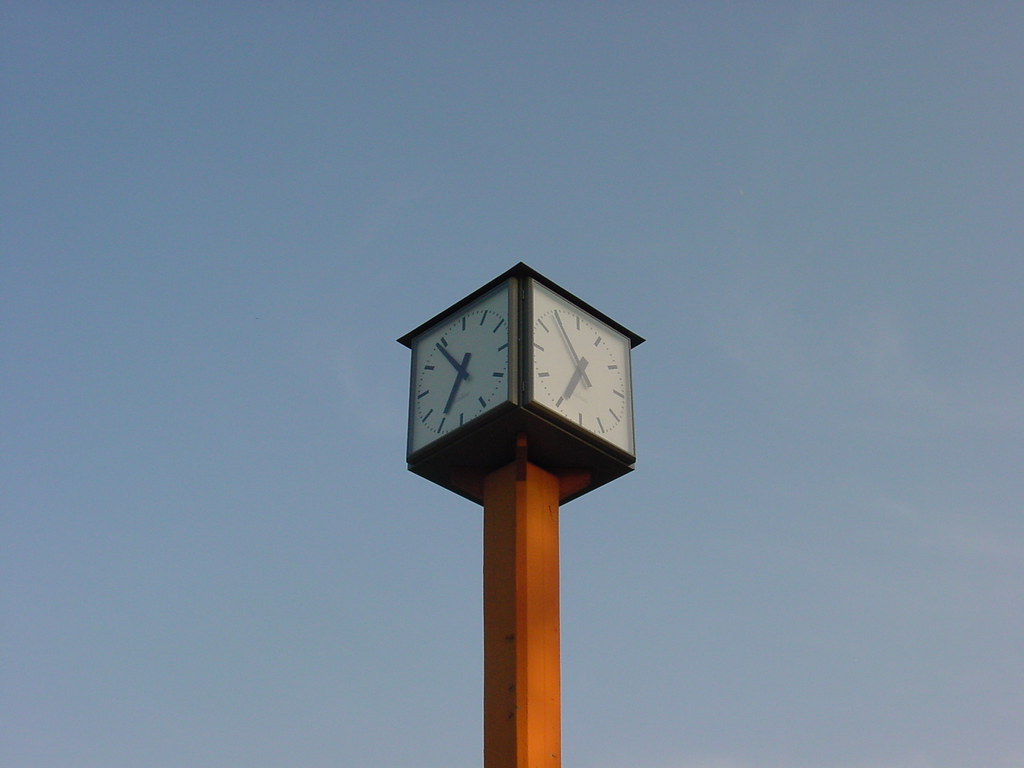This photograph captures a striking clock tower set against a clear, gray-blue sky, bathed in the bright morning sunlight. The centerpiece of the image is a substantial square wooden post or iron beam extending vertically into a cube-shaped clock housing. This clock housing features at least two visible sides, each adorned with a white, square clock face. Both faces are identical, displaying black, analog hands and black markings in place of traditional numbers, with smaller dots demarcating the minutes. The time displayed is precisely 6:54 a.m., evidenced by the short hand pointing to the seven and the long hand nearly reaching the eleven. The clock tower radiates an impression of rustic sturdiness combined with functional elegance, standing tall amidst the serene outdoor ambiance.